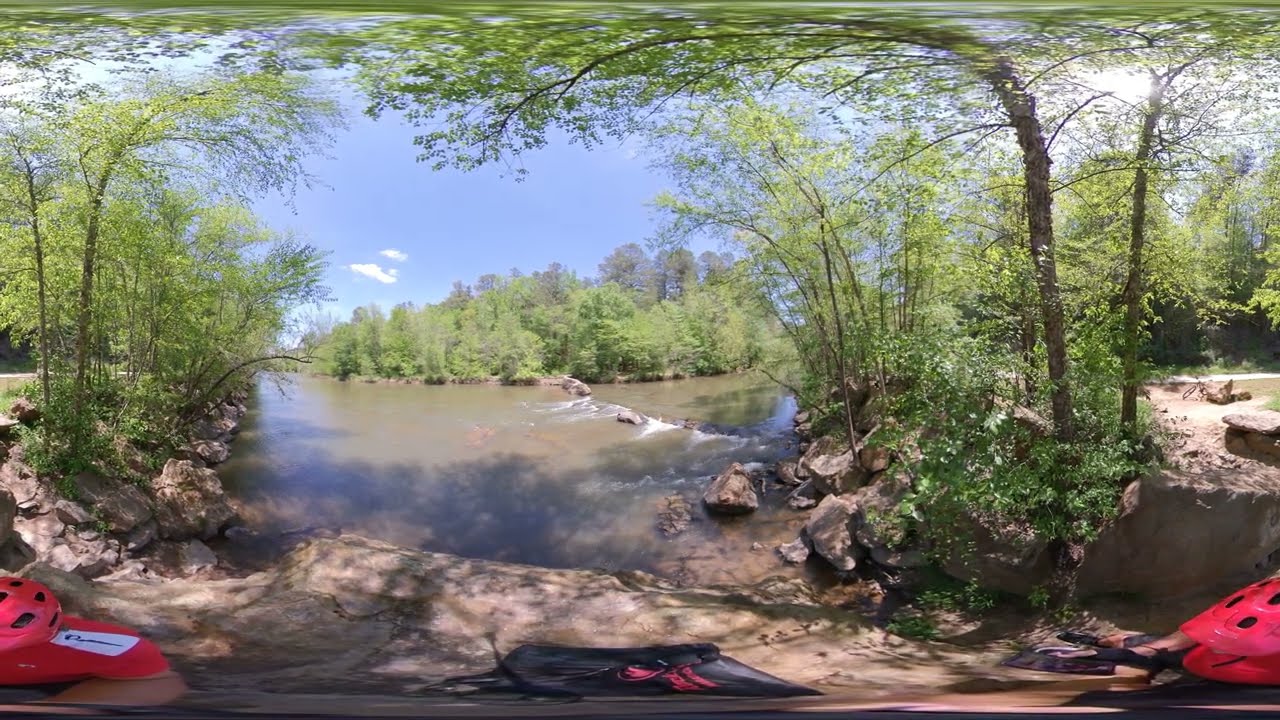This horizontal rectangular photograph, likely taken with an unusual lens, captures a shore area featuring a brown, swampish river or stream flanked by trees. The trees on either side arch toward each other at the top, forming a canopy, while further into the background, the trees regain their upright posture. The image also includes rocky riverbanks and glimpses of the blue sky with sparse clouds above. On the lower left and right corners of the image, there are red objects resembling skidoos or watercraft, suggesting recreational activities such as whitewater rafting. Additionally, there are helmets visible on the lower left and right edges of the image, possibly indicating the presence of people engaged in adventurous water activities, although no individuals are directly visible in the shot. The overall scene conveys a peaceful atmosphere with hints of vigorous activity.